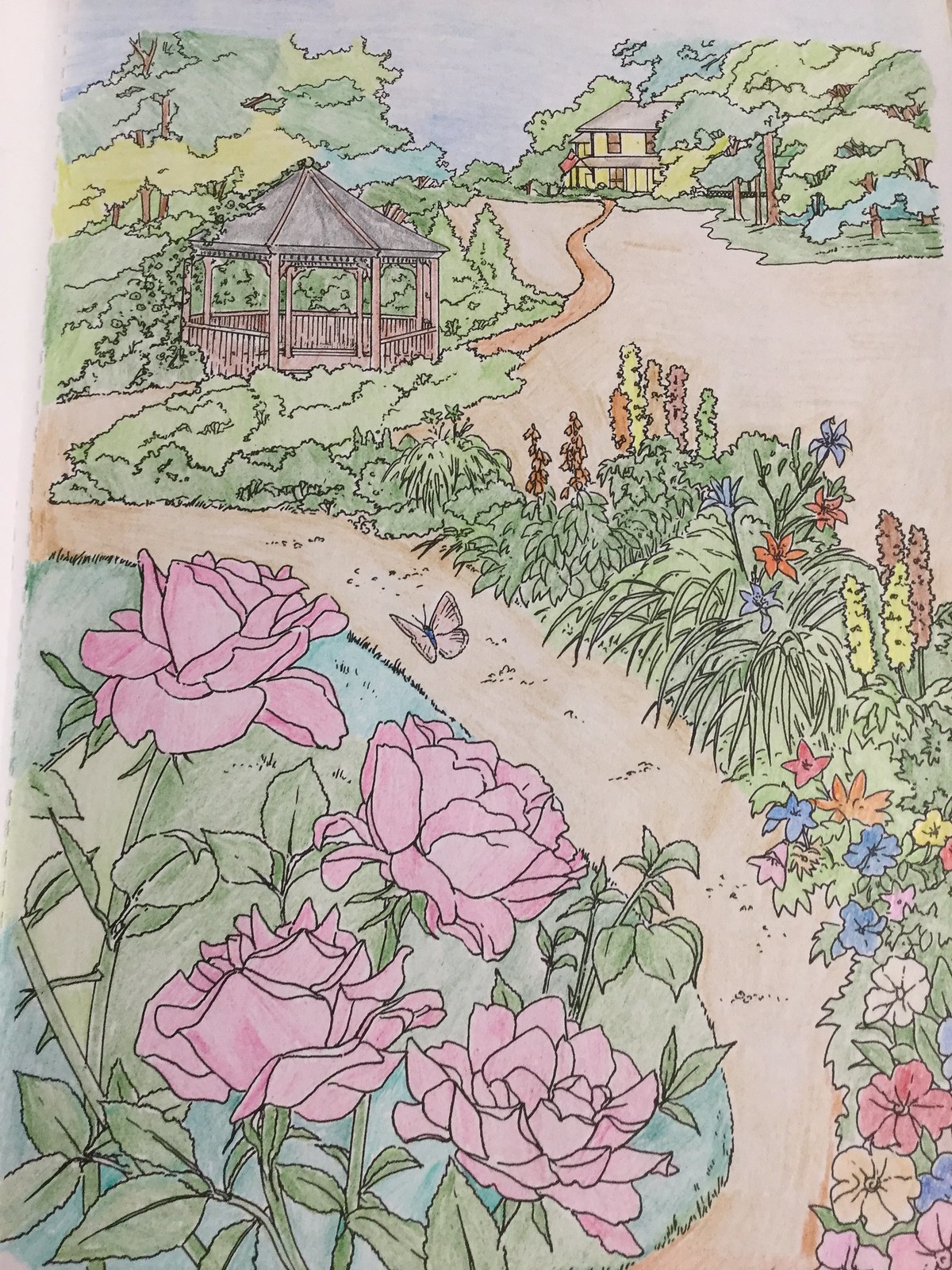The rectangular colored pencil drawing, resembling a page out of an adult coloring book, depicts a vividly detailed garden scene filled with a multitude of colors. The tan path starts from the bottom right and gracefully curves towards the left, flanked by rich greenery, bushes, and a variety of flowers. Prominent among the flora on the bottom left are distinct pink roses, while the right side features more colorful blooms in shades of yellow, orange, blue, and pink. The path meanders through dark and light green grassy areas, guiding the viewer’s eyes to an octagonal brown gazebo surrounded by lush bushes and trees. Continuing towards the upper portion of the image, the path proceeds toward a distant brown house with bright yellow windows nestled among trees displaying various shades of green under a bluish-gray sky.